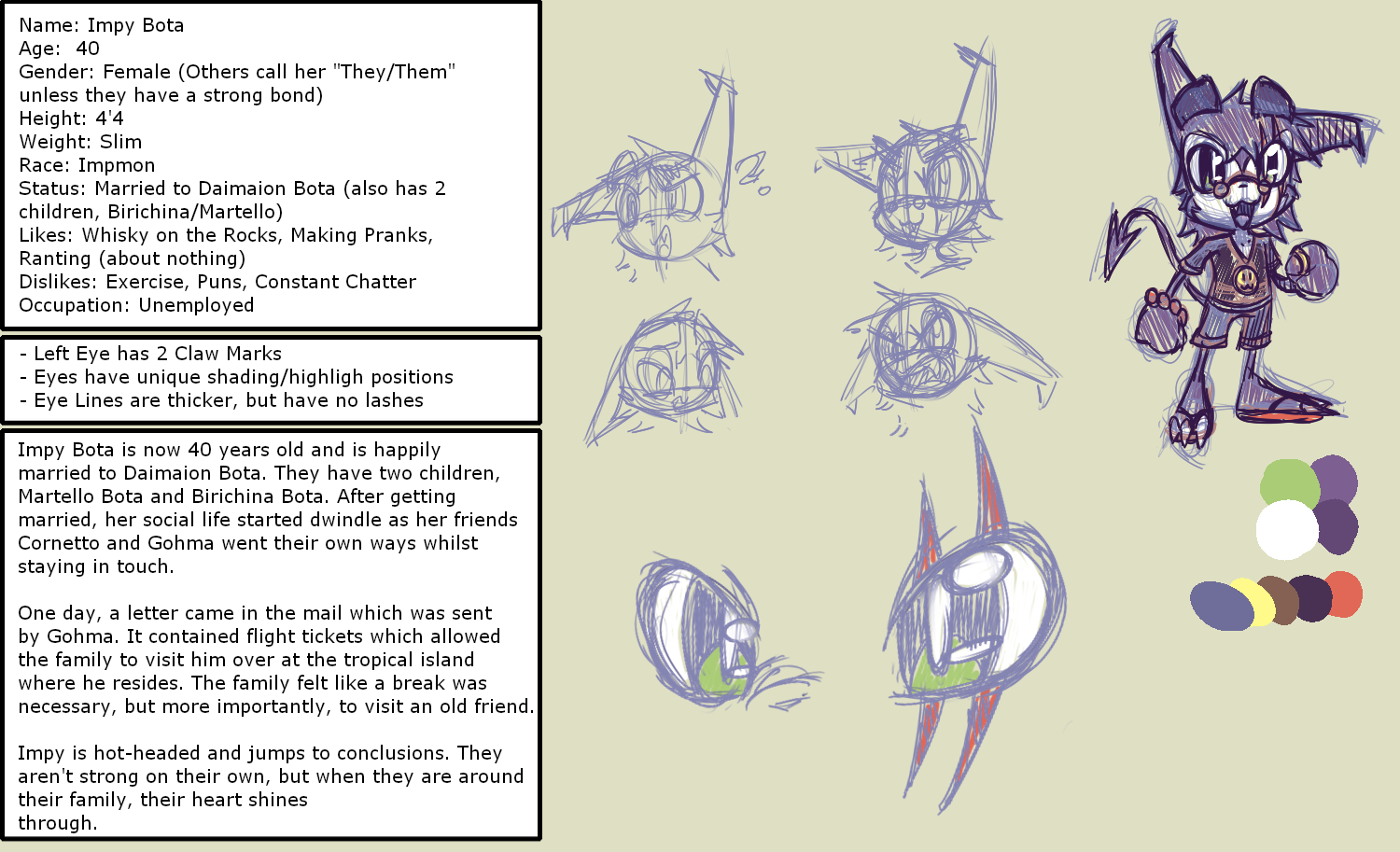This image showcases a detailed character design sheet for a character named Impyboda, also referred to as Impy Bota, likely intended for a video game or animated project. The character is a fox-like creature with notable features including pointy ears, a long devil-like tail, and distinct coloring -- predominantly purple with white facial highlights. 

Impyboda is depicted through several pencil sketches, including four different head representations and a full-body drawing, portraying varying incarnations of the character. The character is wearing a t-shirt and flip-flops. Unique details such as two claw marks over the left eye, specific shading techniques, and thick eye lines without lashes are meticulously noted.

To the left of the sketches, there are three sizable blocks of text providing extensive information about Impyboda: 
- Name: Impyboda (Impy Bota)
- Age: 40
- Gender: Female (referred to as they/them unless there is a strong bond)
- Height: 4'4"
- Build: Slim
- Race: Impmon
- Marital status: Married to Dimayon Bota, with two children named Birichina and Martello.

Accompanying these details, a larger text block presents the backstory and additional character traits. There are also visible color smudges on the sheet (green, white, purple, red, brown, and yellow) hinting at the palette used in the character's creation.